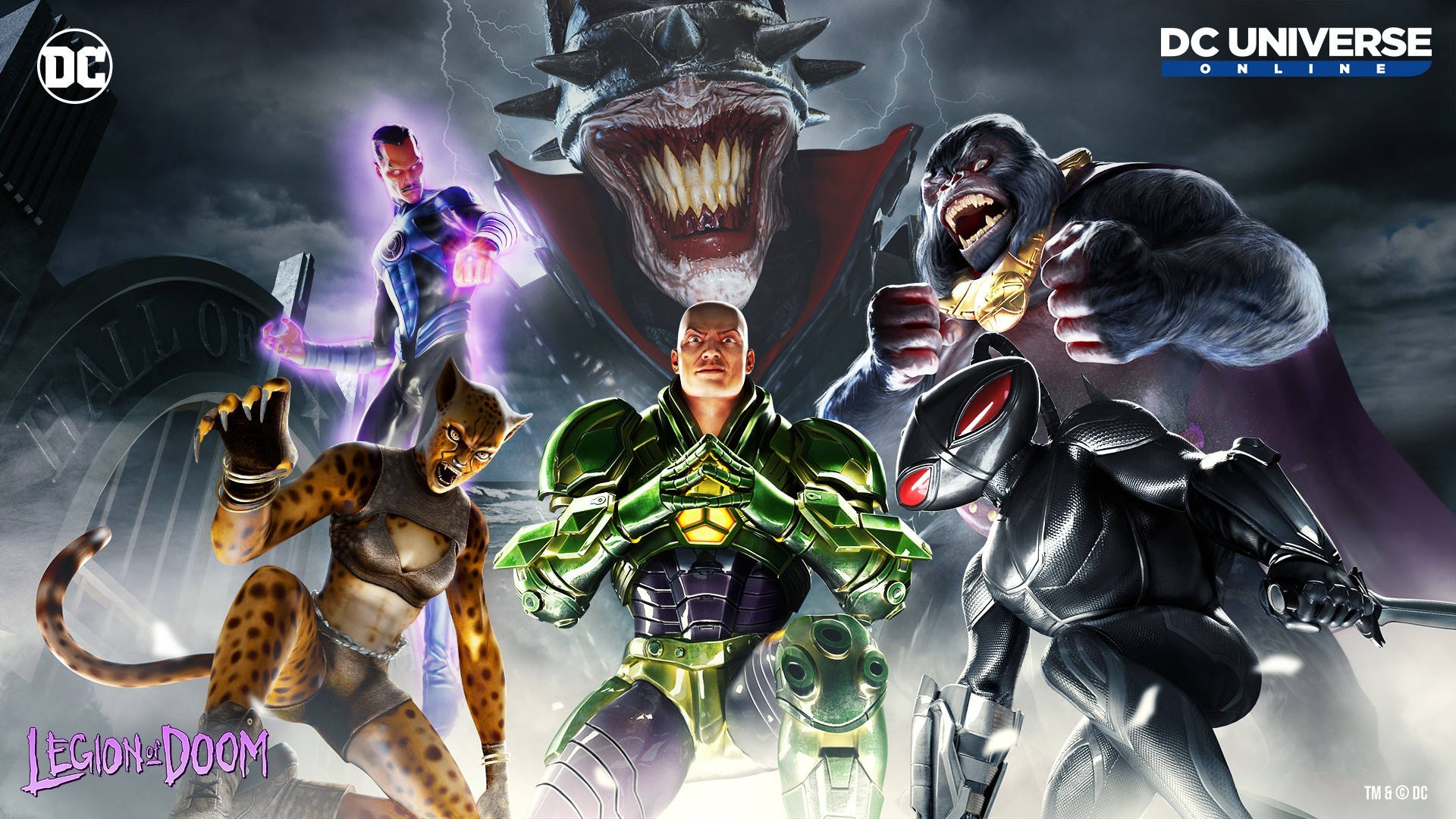In this horizontally oriented image, we see a dynamic assembly of comic-style supervillains. At the top left corner, there's a round DC logo, while the upper right corner is marked with "DC Universe Online" in white letters against a blue background. Dominating the central part of the image is a character in a metallic green and purple suit, with a bald head, and exaggerated, gloved hands. To his left, a snarling, cheetah-like woman bears her fangs threateningly. To his right stands a humanoid ant or bug-like creature equipped with a sword-like appendage extending out of the image's right edge. Above this ant creature looms an ape-like being with a furious expression, bared canine teeth, and muscular arms clutching an indistinct object. Towering over the central figure is a gargantuan beast with sharp, fang-like teeth set into a wide, menacing grin, reminiscent of the Joker from Batman, circled by a spiked collar around its head. The backdrop is filled with dark, ominous clouds, setting a foreboding tone. At the bottom left, the phrase "Legion of Doom" further emphasizes the villainous theme.